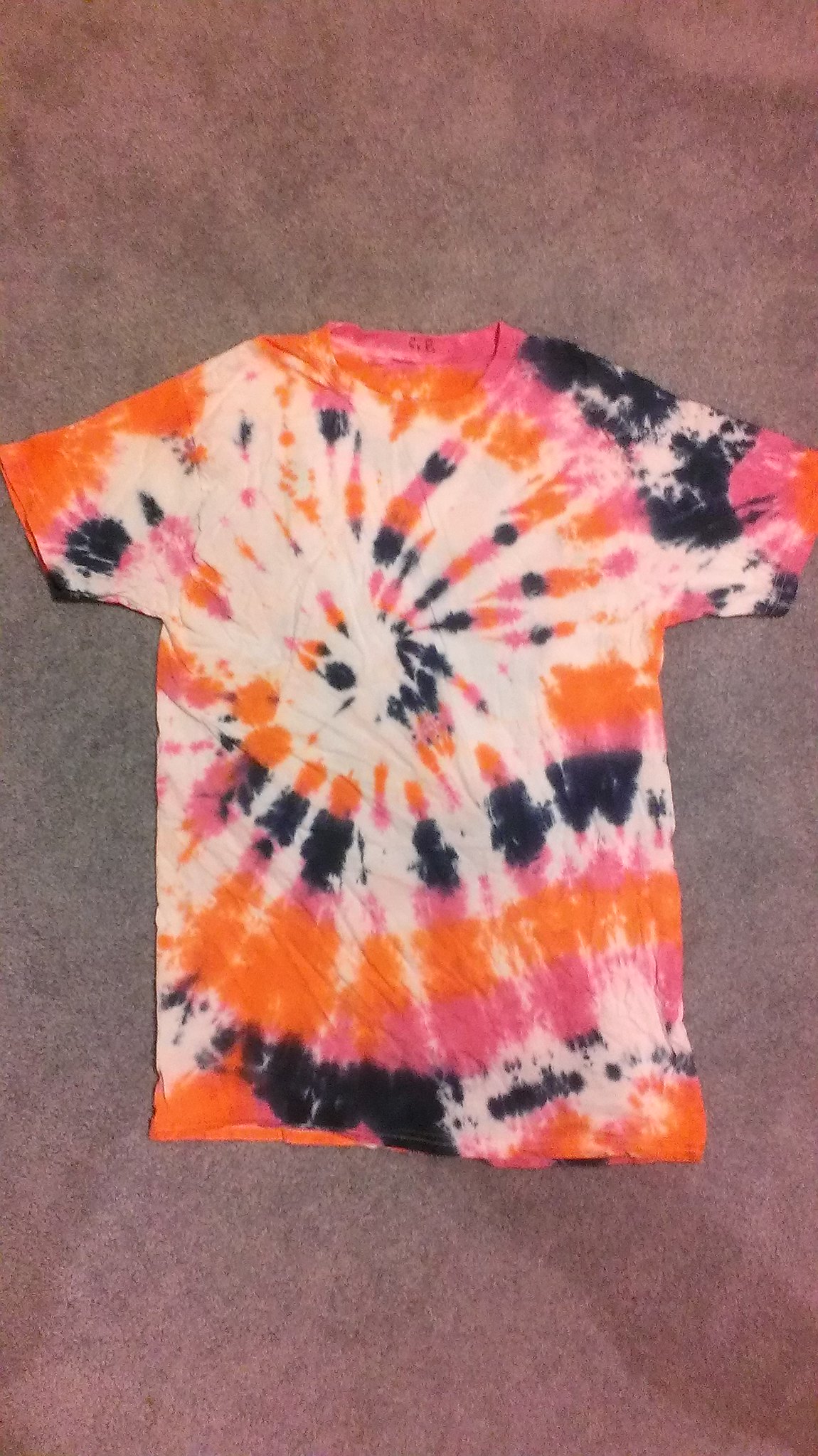This is a detailed photograph of a hand tie-dyed t-shirt, laid flat on a charcoal gray rug. Predominantly, the shirt features vivid shades of pink, orange, and navy blue, with substantial areas of white interspersed throughout, indicative of where it was banded during the dyeing process. The design radiates from the center in a classic swirl pattern, with minor hints of the primary colors concentrated toward the bottom half of the shirt and the right sleeve. The backdrop and overall composition suggest the photo might have been taken to either showcase the tie-dye craftsmanship or to prepare the item for sale.